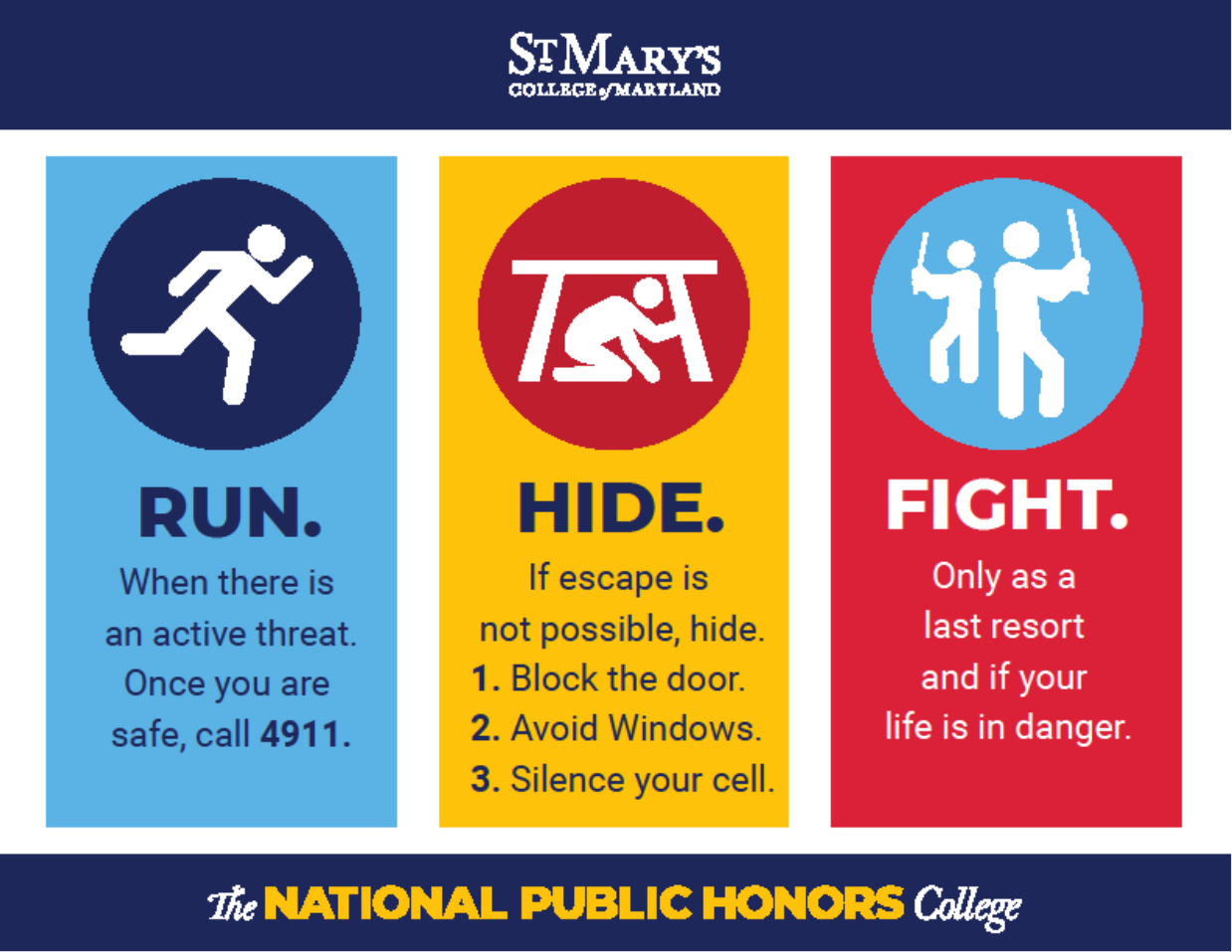This image is a detailed infographic from St. Mary's College of Maryland, designed for active shooter training. At the top, a dark blue banner displays "St. Mary's College of Maryland" in white letters. The bottom banner, also dark blue, reads "THE National Public Honors COLLEGE" in a mix of white and yellow text. Between the banners, there are three rectangular panels, each conveying crucial emergency instructions.

1. The first panel, in light blue, features a white stick figure running inside a dark blue circle and reads "RUN." The accompanying text advises: "When there is an active threat, once you are safe, call 4911."
2. The second panel, in yellow, depicts a white stick figure hiding under a table inside a red circle. The header, "HIDE," is followed by: "If escape is not possible, 1. Block the door, 2. Avoid windows, 3. Silence your cell."
3. The third panel, in red, shows two white figures holding sticks inside a light blue circle. The bold, white text "FIGHT" is explained with: "Only as a last resort and if your life is in danger."

This infographic clearly outlines a three-step process—Run, Hide, Fight—for handling an emergency situation.